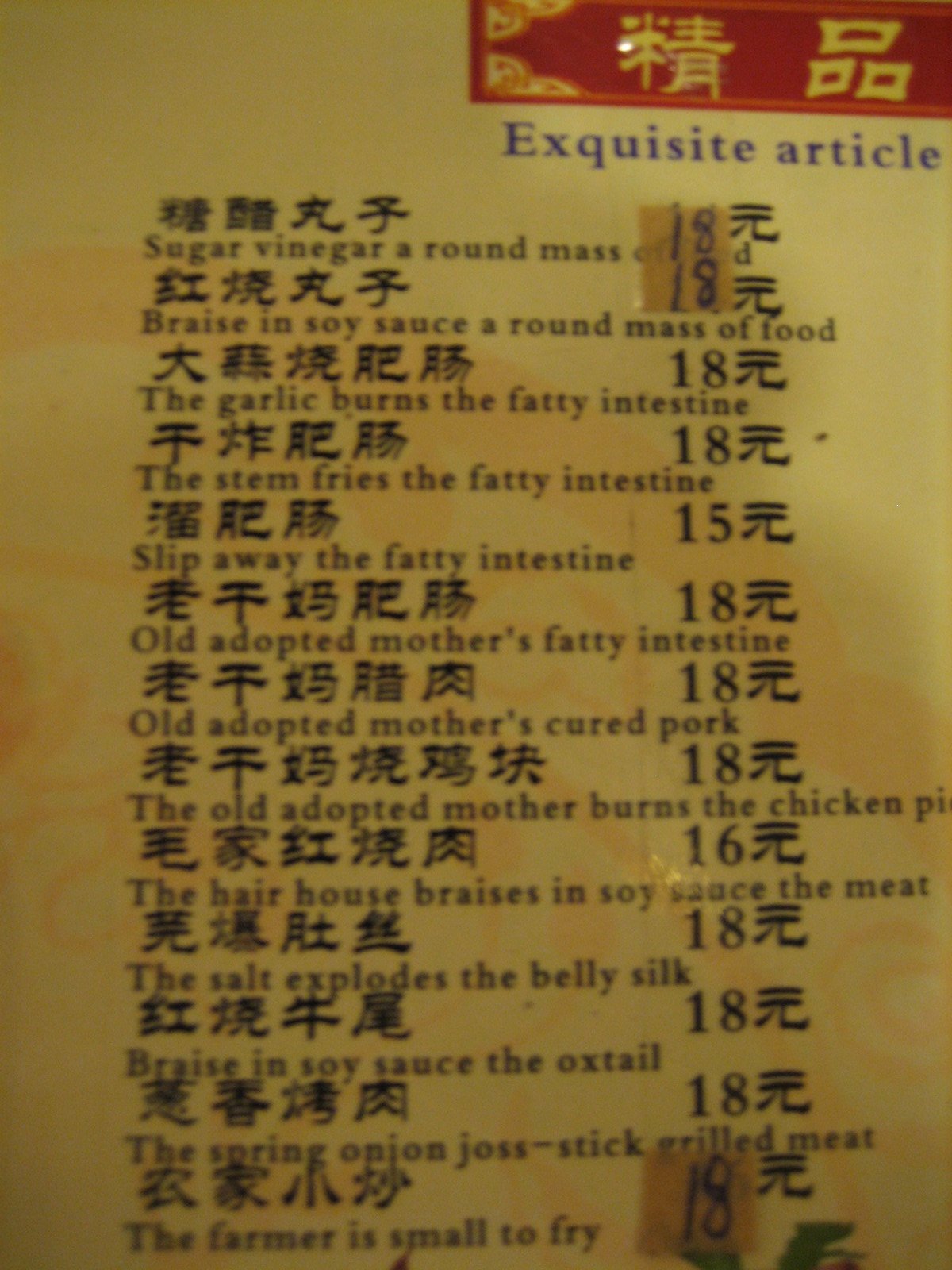The photograph is a close-up shot of a Chinese menu, taken in color, though slightly out of focus and cropped, resulting in an incomplete view of the entire page. The menu appears to be printed on ivory or parchment-colored paper, with a prominent rich red rectangle featured at the top. Within this red rectangle, elegant Chinese characters are printed in gold, flanked by intricate, stylized cloud-like designs in the corners, framed by a slim border running along the bottom.

Beneath this decorative header, the menu presents a series of Chinese dishes, each listed first in Chinese characters followed by an English translation and a corresponding price to the right. While the prices are not the focus here, they predominantly range around 15 to 18 units of currency.

The English translations of the dishes are as follows:

1. Sugar Vinegar Round Mass
2. Braise in Soy Sauce Round Mass of Food
3. The Garlic Burns the Fatty Intestine
4. The Stem Fries the Fatty Intestine
5. Slip Away the Fatty Intestine
6. Old Adopted Mother's Fatty Intestine
7. Old Adopted Mother's Cured Pork
8. The Old Adopted Mother Burns the Chicken
9. The Hare House Braises in Soy Sauce the Meat
10. The Salt Explodes the Belly Silk
11. Braise in Soy Sauce the Oxtail
12. The Spring Onion Joss Stick Grilled Meat
13. The Farmer is Small to Fry

The menu thus offers a tantalizing, if sometimes humorously translated, glimpse into a variety of traditional Chinese dishes.